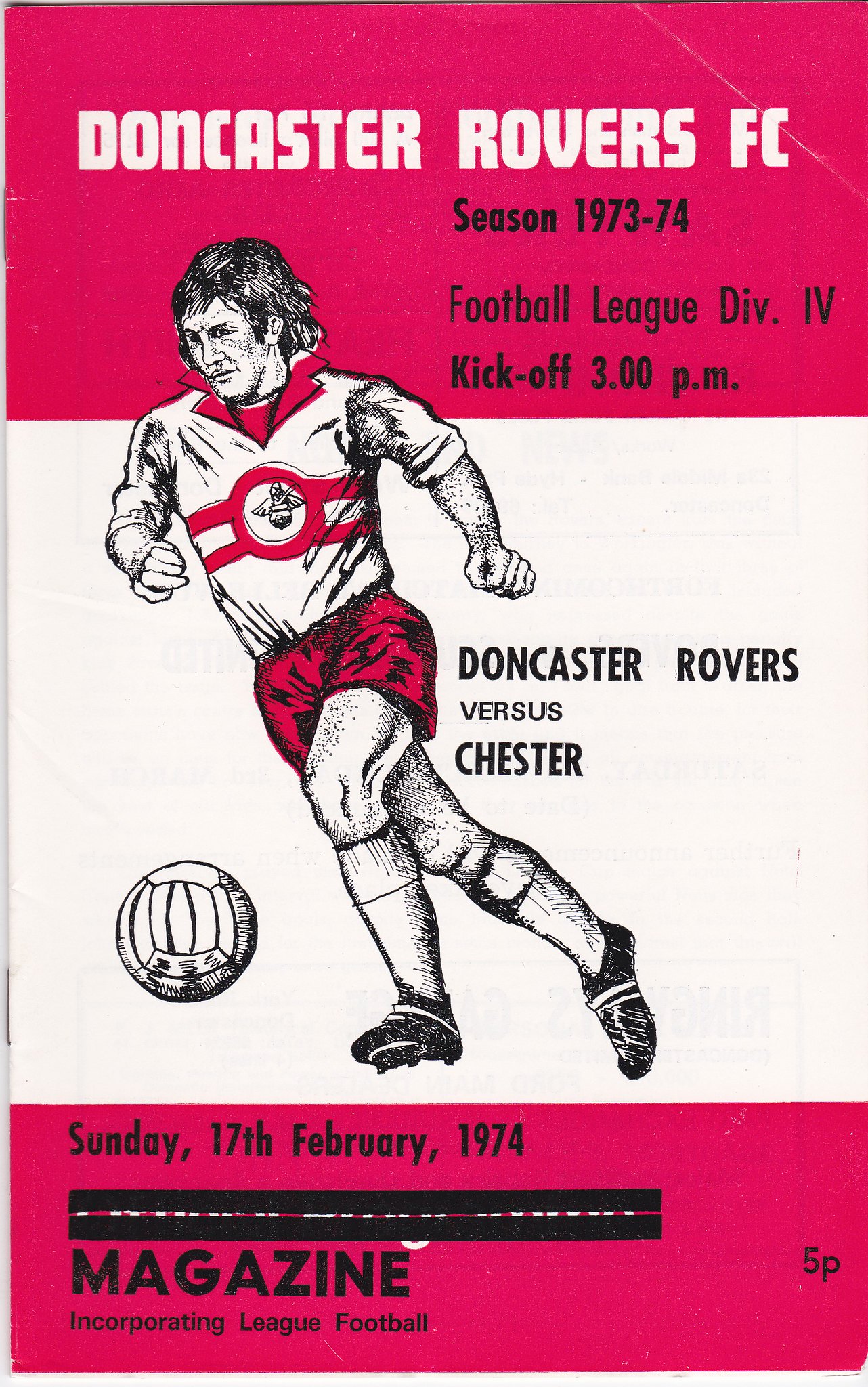This image showcases the cover of an old magazine, specifically a matchday program for a soccer game. The cover is divided into three horizontal sections: the top and bottom thirds are red, while the middle third is white. 

At the top, "Doncaster Rovers FC" is prominently displayed in white text, just above the black text detailing the 1973-74 Season of the Football League Division 4, with a kickoff at 3 p.m. The center section features an illustration of a soccer player wearing red shorts and a white jersey with red stripes. The player's body is mostly within the white middle section, with his head extending into the red top section. He is poised next to a soccer ball, and wears cleats. 

To the right of the player, in black letters, it announces the match: "Doncaster Rovers vs. Chester." The bottom red section of the cover, in black text, notes the date of the match as "Sunday, 17th February 1974," and describes the publication as a "magazine incorporating league football," priced at "5p." Staples are visible along the spine of the booklet. The entire cover is in black and white, further emphasizing its vintage nature.